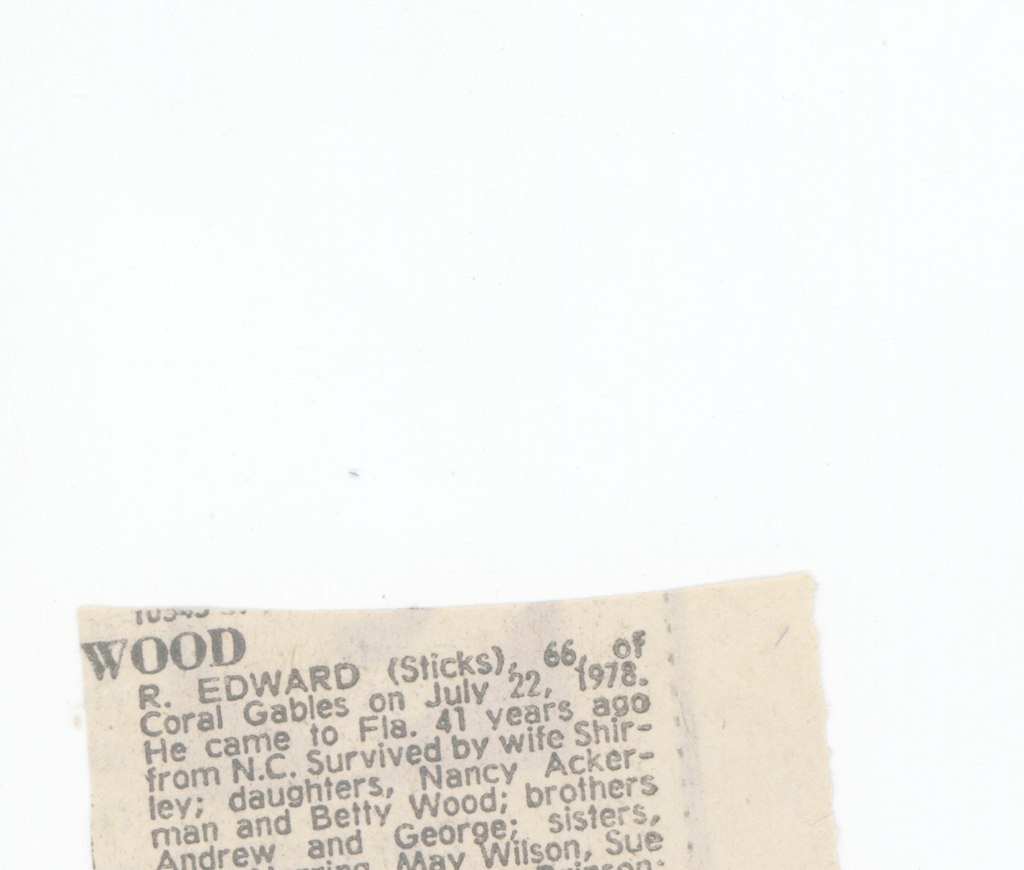The image appears to be a scanned excerpt from an old newspaper obituary column, focusing on R. Edward Stix, 66, of Coral Gables, who passed away on July 22, 1978. The obituary notes that he moved to Florida 41 years ago from North Carolina. He is survived by his wife, Shira Lee, daughters Nancy Ackerman and Betty Wood, and his brothers Andrew and George. The text cuts off before fully listing his sisters, only mentioning names like May Wilson Sue. The paper is visibly aged, exhibiting a yellowish or pinkish tint with gray writing, and the overall image is notably faded. The scan shows the document tilted slightly counterclockwise, with a significant portion of the surrounding area being blank white space.